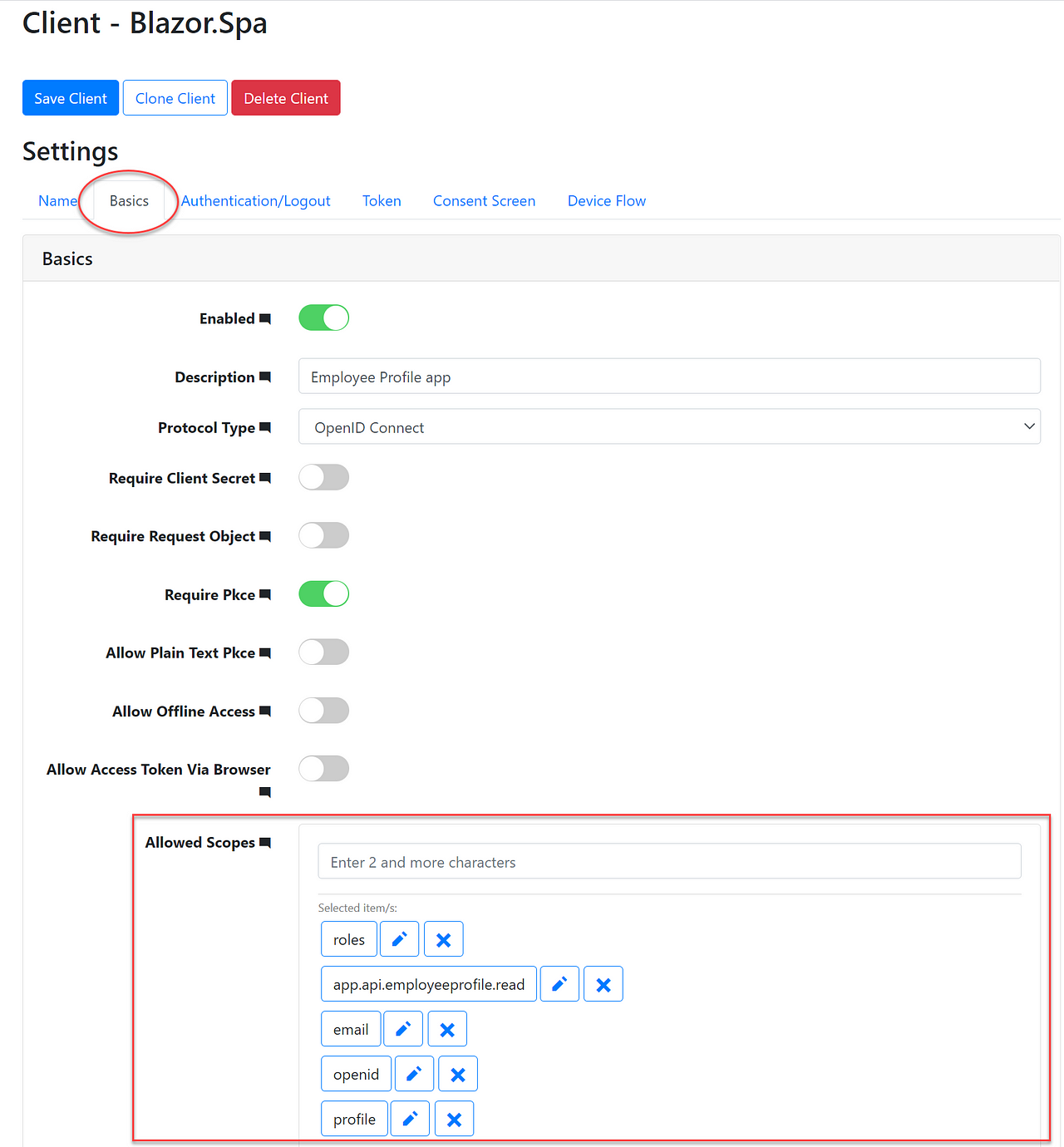The image is a vertical screenshot from a computer or smart device displaying an interface with a white background, likely from a browser. At the top, there's a thin gray horizontal bar, beneath which the bold black text "client-blazor.spa" is displayed.

Below the title, three clickable options are presented: "Save Client" in blue, "Clone Client" in white, and "Delete Client" in red. Under these options, the word "Settings" appears in bold black text.

Further down, a menu of options in blue and black text is visible. The selected option, "Basics," is highlighted in black and circled with a red outline. Other menu items include "Authentication," "Logout," "Token," "Consent Screen," and "Device Flow."

A gray bar with black text labeled "Basics" separates the sections. This area contains several configurations in bold black text, including "Enable," "Description," "Protocol Type," "Require Client Secret," "Require Request Object," "Require PKCE," "Allow Plain Text PKCE," "Allow Offline Access," and "Allow Access Token via Browser." Toggles for "Enabled" and "Require PKCE" are both switched on.

At the bottom of the interface, surrounded by a red outline, is a box labeled "Allowed Scopes." Inside the box, text prompts the user to "Enter two or more characters," with various selectable options listed below.